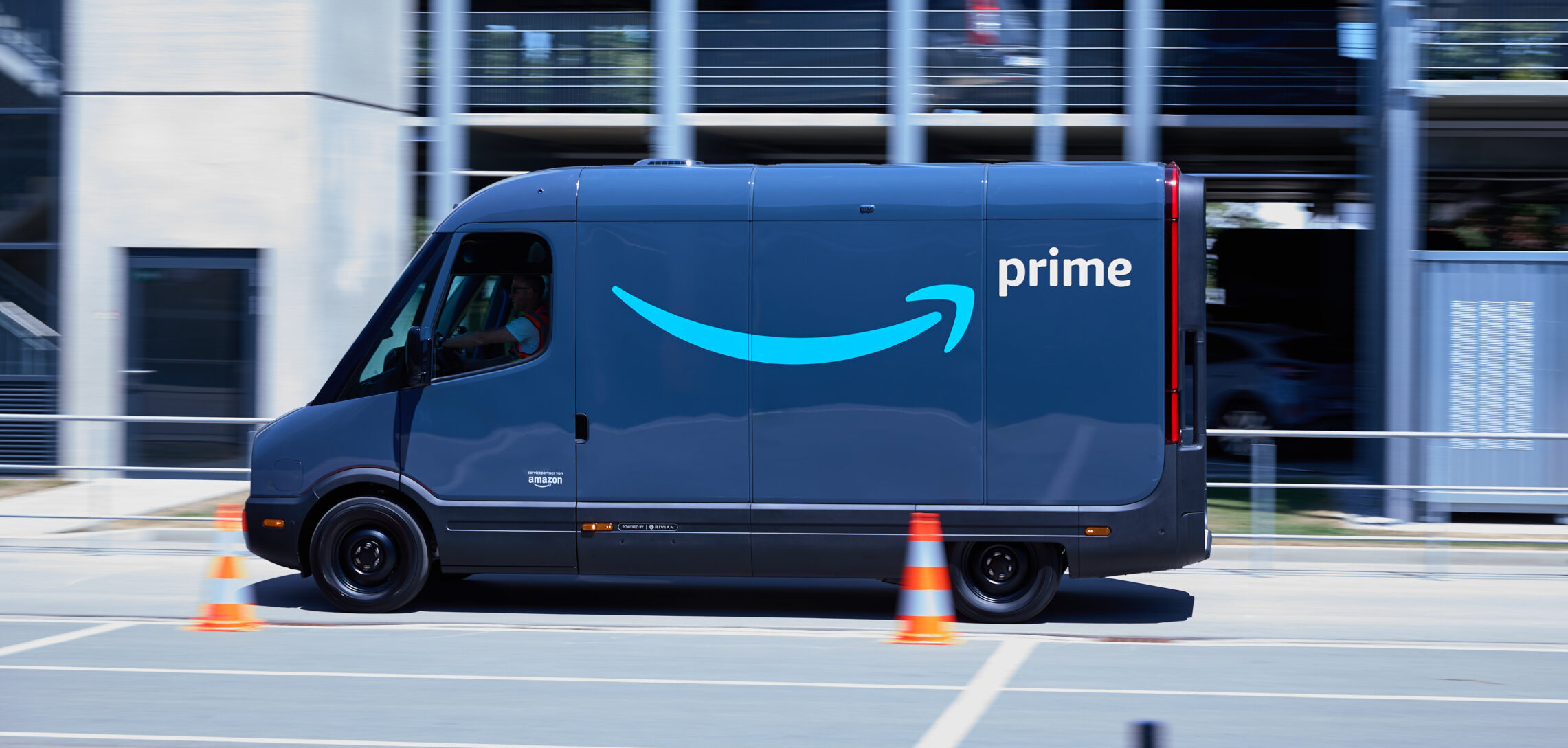In this dynamic image, an Amazon delivery van, likely one of the newer Rivian models, is captured in motion, with most surrounding elements appearing blurred due to its speed. The van itself, however, is sharply defined. It sports the characteristic Amazon Prime logo, featuring the iconic arrow/smile symbol pointing towards the "Prime" text on the right side, near the top of the vehicle. The van is painted in Amazon's signature blue, and despite the motion blur of the background, its black tires and all-black hubcaps are clear and prominent.

The setting appears to be a street bordered by a multi-layered parking complex, with its gray pavement marked by white lines. Some traffic cones, though blurred, can be seen beside the van, adding to the sense of movement. Through the van's windows, a driver is faintly visible, further emphasizing the vehicle's in-use state. In the background, partially obscured yet noticeable, a shadowy parked vehicle is discernible within the parking structure. The overall composition captures the essence of a bustling delivery scene in an urban environment.